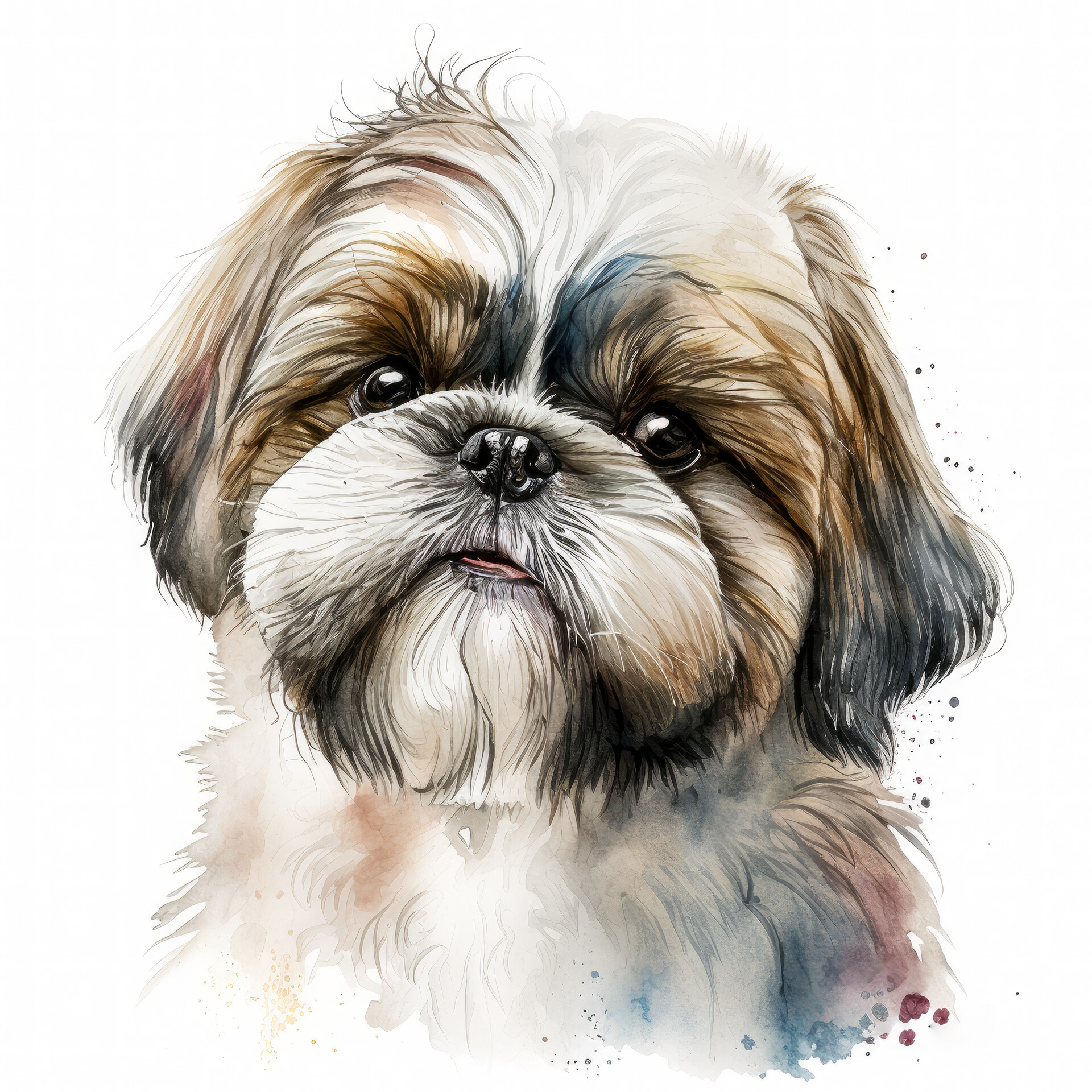This detailed watercolor painting captures the charming essence of a small, friendly Yorkie. The dog’s well-maintained fur is a mix of dark gray, brown, and white, featuring well-trimmed fur free from the characteristic overgrowth around the eyes. The artist cleverly incorporates elements of abstraction with strokes of blue and red in the lower detail section, around the chest area, adding a unique visual interest. The eyes of the Yorkie are exceptionally lifelike, large, and brown, evoking a sense of realism reminiscent of a photograph. Additional hues of black, particularly in the ears, offer a striking contrast. The painting highlights the dog's adorable features, including its bright black nose and tongue peeking out slightly, framed by floppy, fur-covered ears tinged with dark bluish tones. Dabs of red color around the outer edges of the artwork further enhance its vivid appearance, making the little Yorkie look both lively and affectionate.